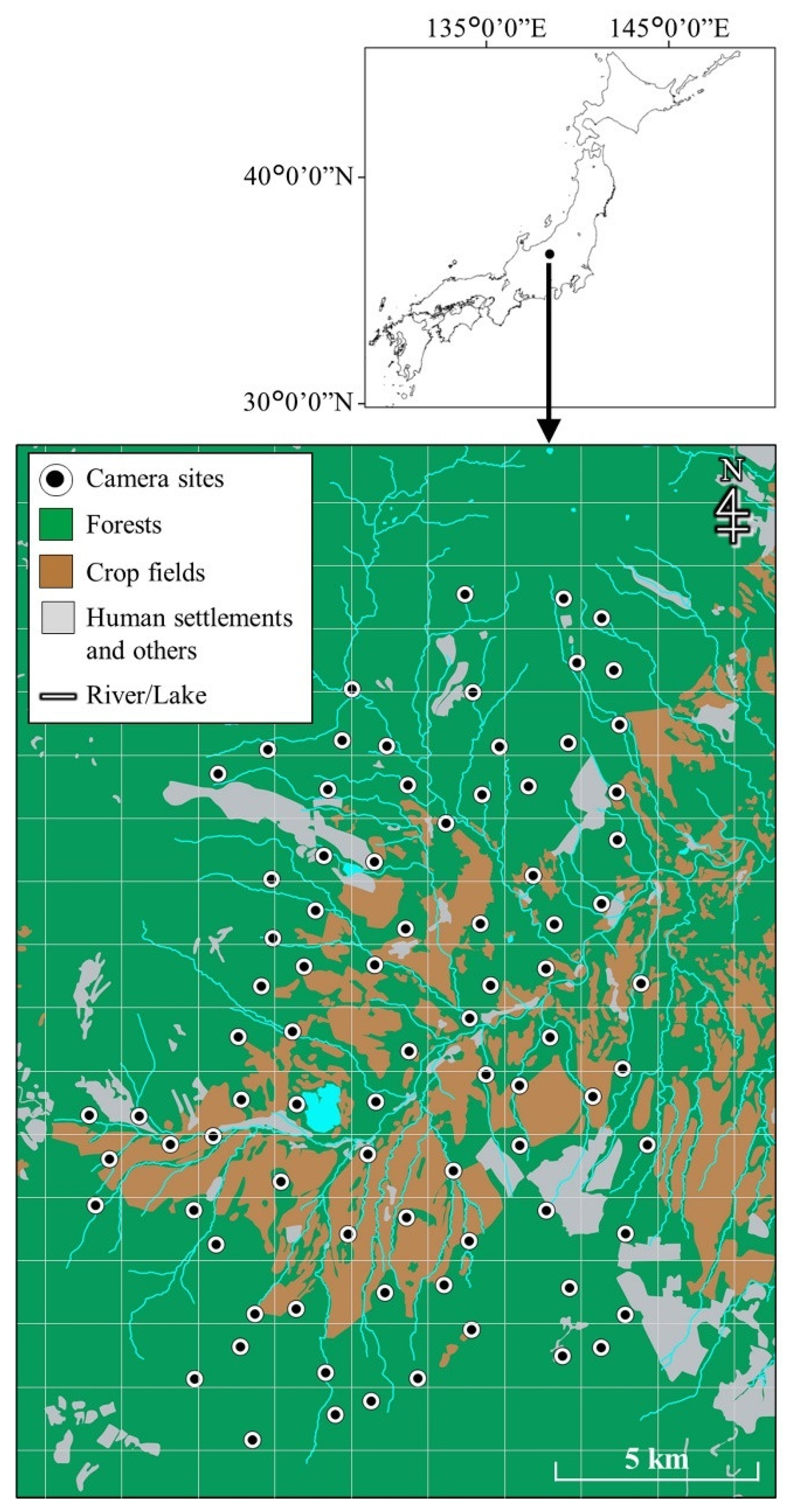The image displays a detailed map with a green background overlaid with white horizontal and vertical grid lines. Located in the upper left-hand corner is a white legend, which provides symbols and their meanings: a black dot within a circle symbolizing camera sites, a green square for forests, a brown square denoting crop fields, a gray square representing human settlements, and a line for rivers and lakes. 

At the top, there is also a smaller inset map of Japan with coordinates (30°00' N, 40°00' N, 135°00' E, 145°00' E) marked in degrees. A large, dark arrow from this inset map points downwards towards the main, larger map below. This main map highlights various regions in accordance with the legend, showing camera placements with black dots, expanses of green and brown indicating forests and crop fields respectively, light blue lines marking the rivers, and gray zones showing human settlements. In addition, the bottom right corner features a scale denoting five kilometers for distance measurements, and the top left displays a directional marker with 'N' for north.